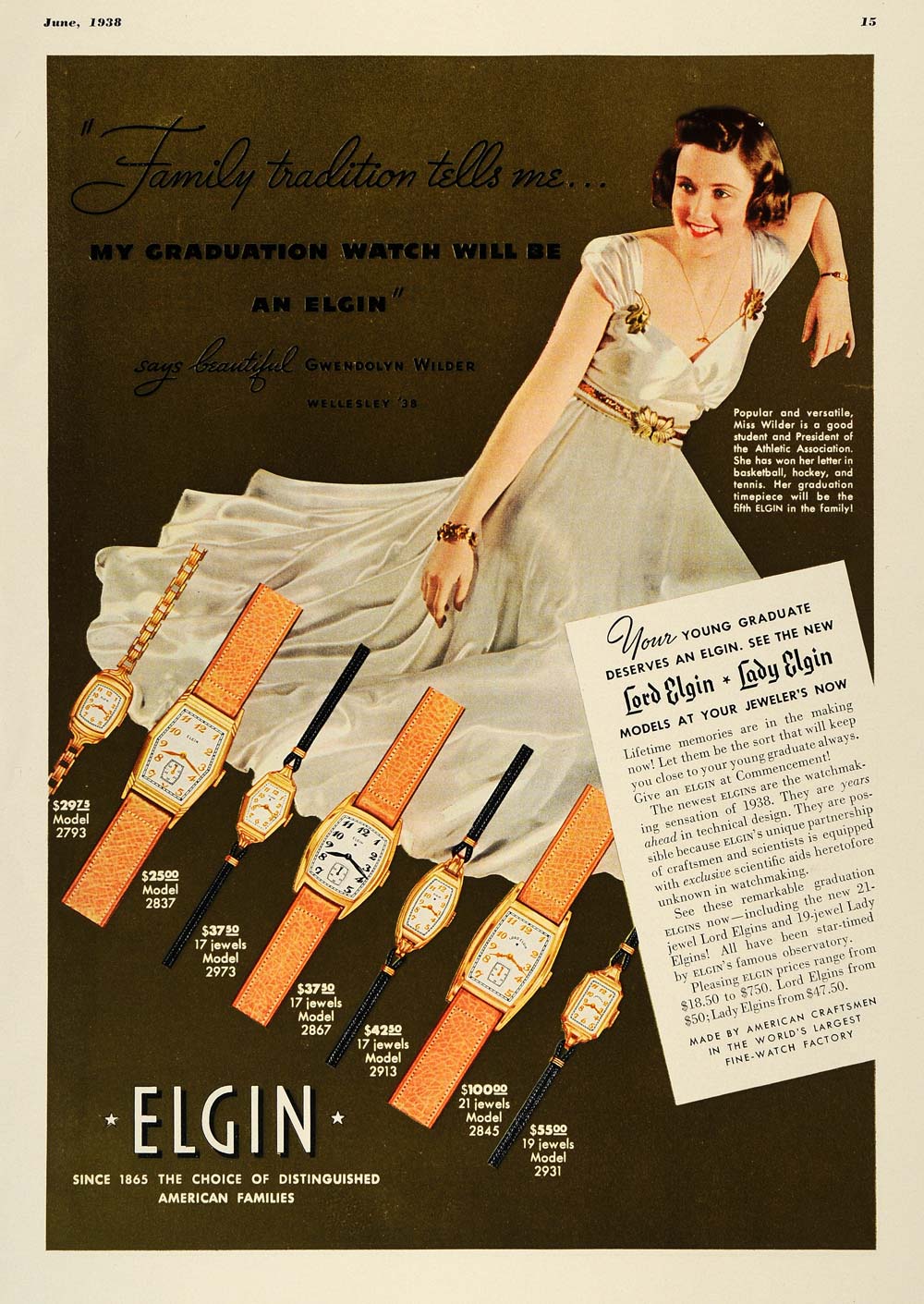This advertisement, possibly from a 1938 or 1958 magazine, showcases Elgin Watches, known since 1865 as the choice of distinguished American families. Occupying a full-color, vertical page, the ad features a white woman with brown hair, elegantly dressed in a shimmery, low-cut white satin gown, adorned with golden accents, including a golden belt, and wearing an Elgin watch. She is posed facing left, with a backdrop displaying an assortment of seven different Elgin women's watches along one side. The tagline at the top reads, "Family tradition tells me my graduation watch will be an Elgin," and at the bottom, it promotes both "Lord Elgin" and "Lady Elgin" models, encouraging readers to visit their jeweler. The setting implies sophistication and heritage, targeting those seeking a timeless graduation gift.